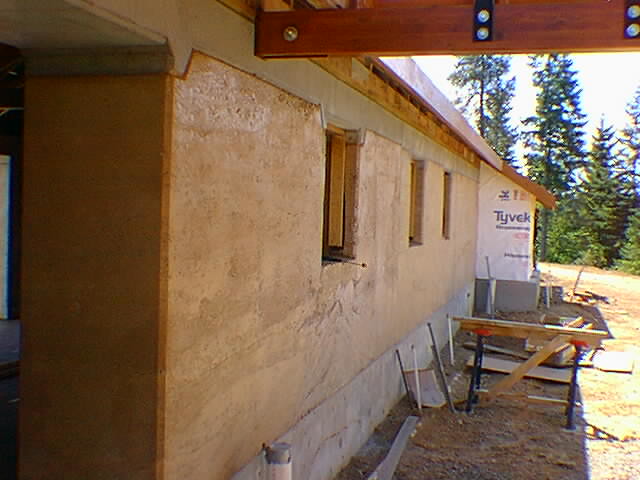The photograph depicts a construction site of what appears to be a single-story building, possibly a house, barn, or stable. The structure is situated in a clearing surrounded by tall, green trees under a whitish-blue sky. The walls of the building are unfinished, with tan plywood covering and a gray cement foundation. There are three vertical rectangular window cutouts along the side wall, still devoid of glass. A wooden beam extends out from the upper part of the structure, suggesting the future addition of a porch. In the distance, a section of the wall is covered with a white sheet bearing the name "Tyvek" in blue letters, indicating ongoing construction. The foreground features a dirt lot with patches of dead grass and a pipe protruding from the ground. The image appears to have been taken at an angle, showcasing the length of the building and the surrounding forest setting.